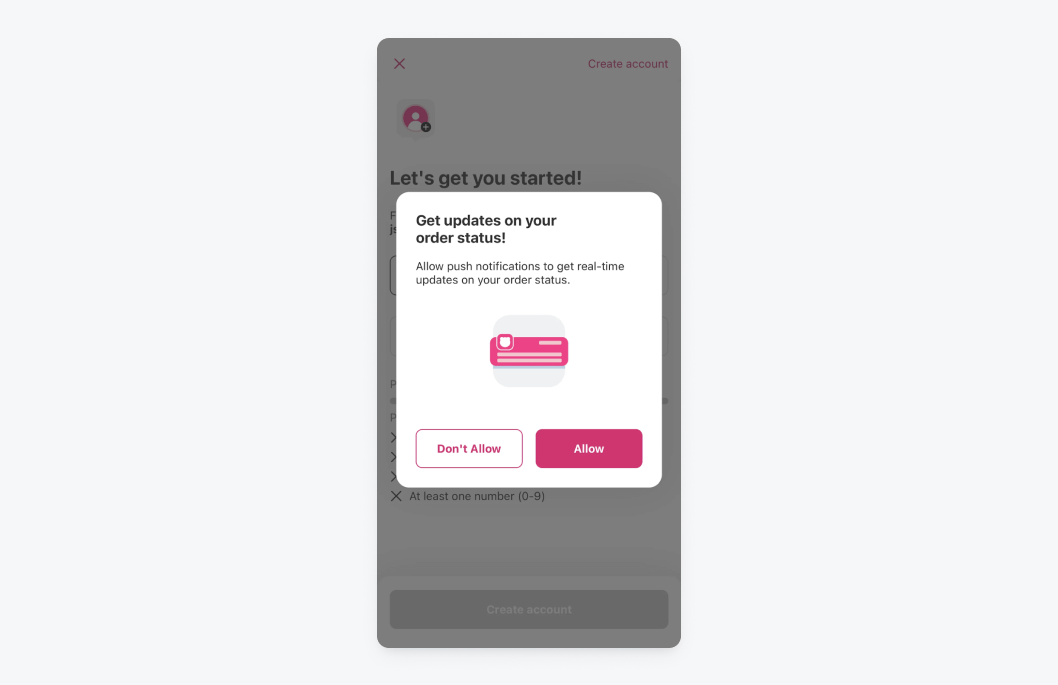The image depicts a screenshot with a grayed-out background, framed within a larger gray box. At the top, there is a prominent pink 'X' icon. Below this, a pink circle contains a white cartoonish person icon, followed by a gray and white plus sign symbol. In pink text, the phrase "Create Account" is displayed. 

Beneath this heading, black text states, "Let's get you started." A white pop-up window overlays the grayed-out background, featuring a smaller white box with black text that reads, "Get updates on your order status." An explanation follows: "Allow push notifications to get real-time updates on your order status," accompanied by a pink and white credit card-like icon.

Below the explanatory text, two buttons are present: a white and pink box labeled "Don't Allow" and another white and pink box labeled "Allow." The "Allow" button is pre-selected. 

At the bottom of the image, a gray box with white font reads "Create Account." Although the underlying grayed-out image appears to contain potential instructions for setting up a password, no other significant text or elements are present. The image is noted for its high visual quality, with clear, legible text and no signs of pixelation or blurring.